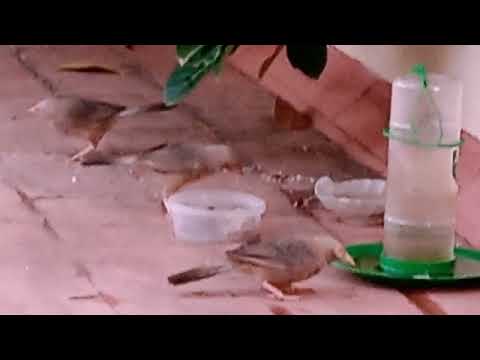The image captures an outdoor feeding and watering area for birds, set on a terracotta-colored surface that resembles red brick. In the right-hand side of the image, there is a clear plastic bird feeder with a green water reservoir at the bottom. A brown bird is seen drinking from this reservoir. On the left side, another brown bird with tan-tipped wings and a brown tail is eating from one of the two white plastic containers placed on the ground, which are meant for seeds. Additional feed appears scattered on the ground near the containers. The background features three green leaves positioned in the upper middle, indicating the area is under some foliage, likely a plant or shrub. The scene unfolds on a sunny day, though the image has a reddish overtone and is slightly blurry, further enclosed by a black header and footer.